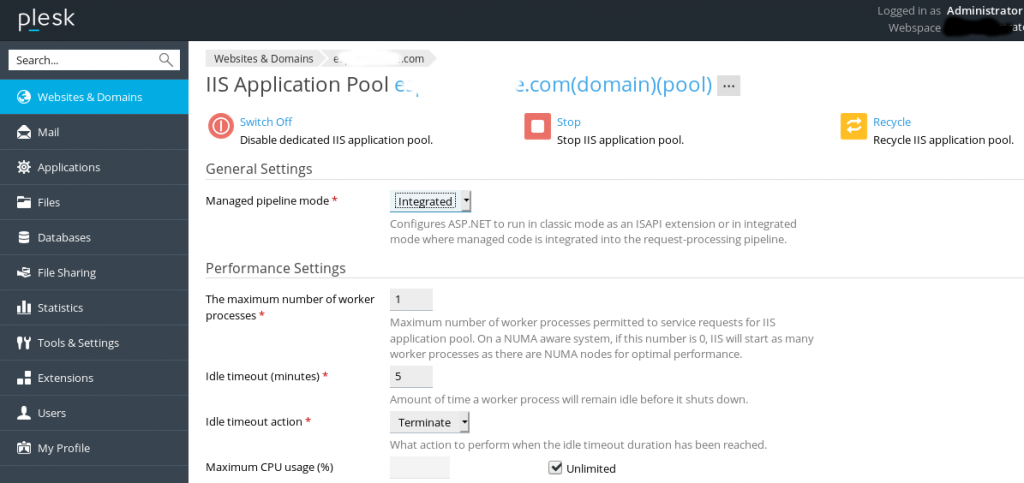This is a detailed view of a Plesk web interface page, showcasing the "Websites & Domains" section. The overall theme is a white font set against a black background. Along the left-hand side, there is a vertical menu featuring various sections: 

1. **Websites & Domains** (highlighted in blue with a globe icon),
2. **Mail**, 
3. **Applications**, 
4. **Files**, 
5. **Databases**, 
6. **File Sharing**, 
7. **Statistics**, 
8. **Tools & Settings**, 
9. **Extensions**, 
10. **Users**, 
11. **My Profile**.

These menu items are all displayed in white font against the black background.

On the main panel to the right, the "Websites & Domains" section is active. It includes various controls and settings for an IIS application pool. The top section displays a domain placeholder "**E***E.com**, indicating partial masking of the actual domain name. The label indicates this is for the **domain** and **pool**, accompanied by a gray square with three dots for additional options.

Key interactive buttons are displayed prominently:
- **Switch Off**: A red circle with blue text that allows users to disable the dedicated IIS application pool.
- **Stop**: A red square with blue text to stop the IIS application pool.
- **Recycle**: A yellow square with blue text and arrows pointing both ways, offering the option to recycle the IIS application pool.

The page continues with settings tabs for:
- **General Settings**: 
  - Managed Pipeline Mode, displayed as "Integrated" in a drop-down box with a description explaining options for running ASP.NET in classic or integrated modes.
- **Performance Settings**: 
  - Maximum number of worker processes set to 1 by default, with details on US application pools and Pneuma-aware systems.
  - Idle Timeout, set to 5 minutes, specifies the duration a worker process remains idle before shutting down.
  - Idle Timeout Action, set to "Terminate," defines the action performed after the idle timeout duration.
  - Maximum CPU Usage, which has a blank field with an option to check a box labeled "Unlimited."

Overall, the interface allows users to manage various operational aspects of their websites and domains efficiently through clearly labeled sections and intuitive control elements.